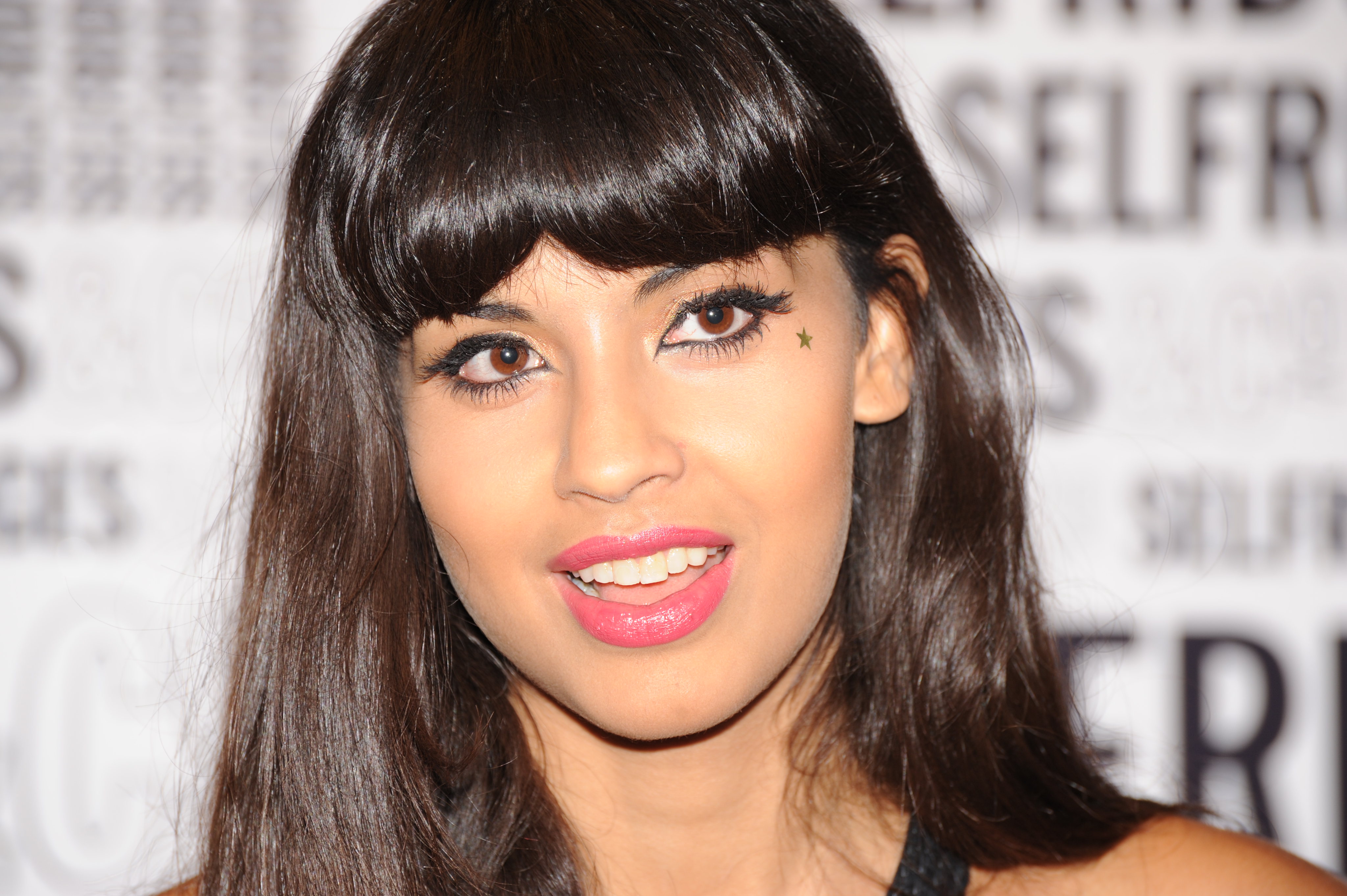The photograph showcases a beautiful young woman with dark, shoulder-length hair and bangs. She is wearing pink lipstick with her mouth slightly open, revealing her teeth. Her captivating eyes, adorned with eye makeup, are brown in color, and she has a small, distinctive beauty mark just below the corner of her right eye. In addition, there is a tiny golden star near her left eye. The woman is tilting her head towards her right (the left side from the viewer's perspective) and is dressed in something black, with a visible strap at the bottom of her neck. She stands against a white background filled with black text of varying sizes, though the words are mostly blurred and illegible except for a few scattered letters like "S," "E," "L," "F," "R."